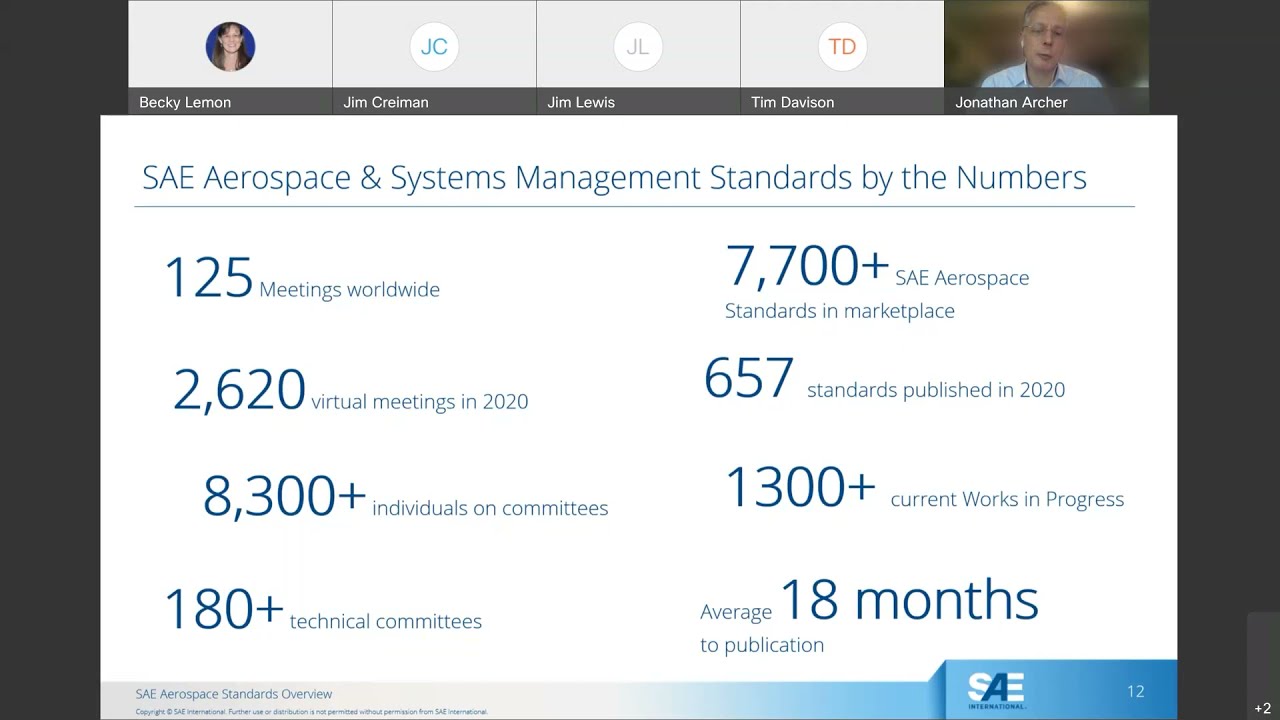This detailed screenshot from a Zoom call depicts a meeting centered around a slideshow presentation titled "SAE Aerospace and Systems Management Standards by the Numbers." At the top of the screen, five participants are listed: Becky Lemon, Jim Cramon, Jim Lewis, Tim Davidson, and Jonathan Archer. Jonathan Archer has his video on, while the others either display their initials or profile pictures.

The slideshow being presented features a white background with light blue lettering and includes various facts and figures about aerospace standards. Notable metrics include "7,700+ SAE Aerospace Standards in the Marketplace," "18 months average to publication," "125 meetings worldwide," "2,620 virtual meetings in 2020," "8,300+ individuals on the committees," "180+ technical committees," "657 standards published in 2020," and "1,300+ current works in progress."

The bottom left-hand corner of the screen shows a trademark symbol, further adding to the professional look of the presentation. This comprehensive visual captures a detailed moment of a professional discussion regarding aerospace standardization.